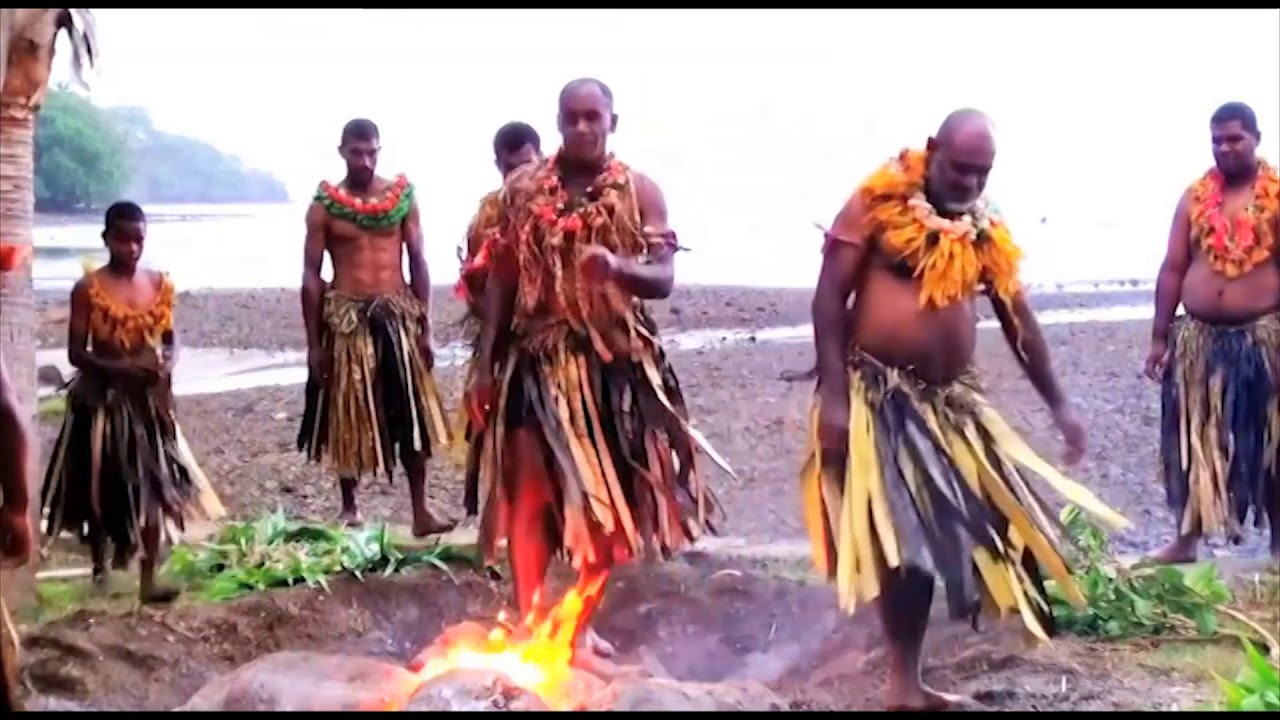The photograph captures a vivid scene of six native islanders, predominantly men with one woman, gathered on a beach in a tropical setting, showcased against the expansive backdrop of the ocean on an overcast day. All individuals are adorned in traditional attire, donning skirts made of palm leaves and colorful flower leis around their necks. Their dark skin glows in the natural light, reflecting their rich cultural heritage. The group is encircling a fire pit set in the sand, where one man appears to be performing a fire-walking ritual, with another seemingly just having completed it, moving away from the focal point. This ceremonial dance, filled with a mix of seriousness and joy, is highlighted by the partial coverage of their chests with the flowery wreaths. Palm trees and additional vegetation punctuate the background, accentuating the cultural and natural essence of the scene. The woman, distinct on the far left, has her breast partially obscured by her wreath, adding to the authenticity and intricate detail of traditional clothing in this captivating moment.